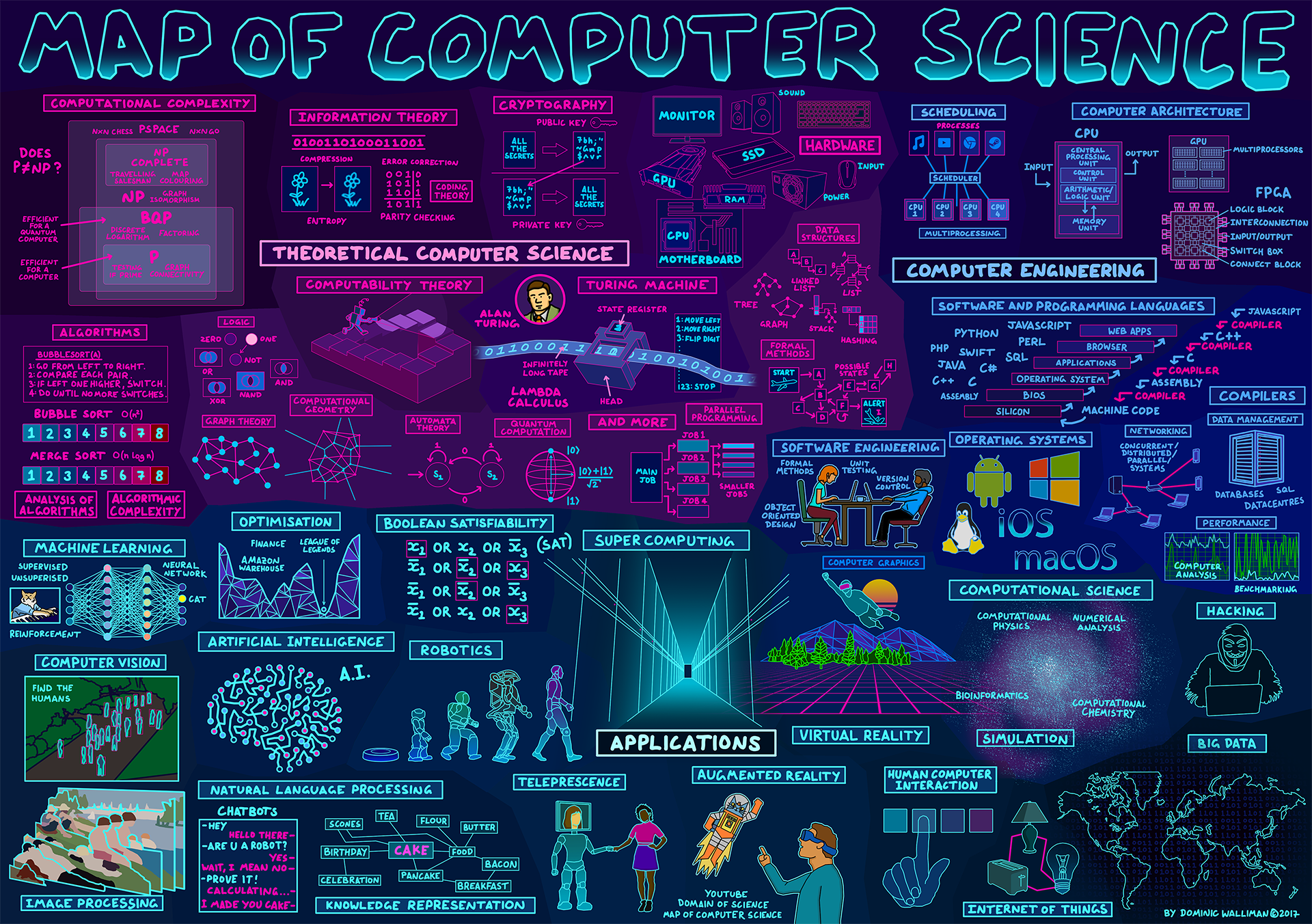The image frame is horizontally rectangular and features a predominantly dark background, transitioning from deep black to dark blue hues. Along the top of the frame, there is a bright neon teal outline forming the words "Map of Computer Science." The central and upper portion of the frame showcases a cluster of information related to theoretical computer science, all displayed in vivid neon colors. 

A horizontally centered, nearly rectangular section extending to just right of the middle is illuminated in bright neon pink. Within this section, terms such as "Computational Complexity," "Information Theory," "Cryptography," and "Monitor Hardware" are clearly listed, accompanied by various images and diagrams.

The remaining portion of the frame is filled with a teal green neon highlighting more applied areas of computer science. Here, we see categories like "Machine Learning," "Optimization," "Boolean Satisfiability," "Supercomputing," "Natural Language Applications," "Computer Engineering," and "Computational Science." Various images and explanatory diagrams are scattered throughout, providing a comprehensive visual map of the field of computer science.